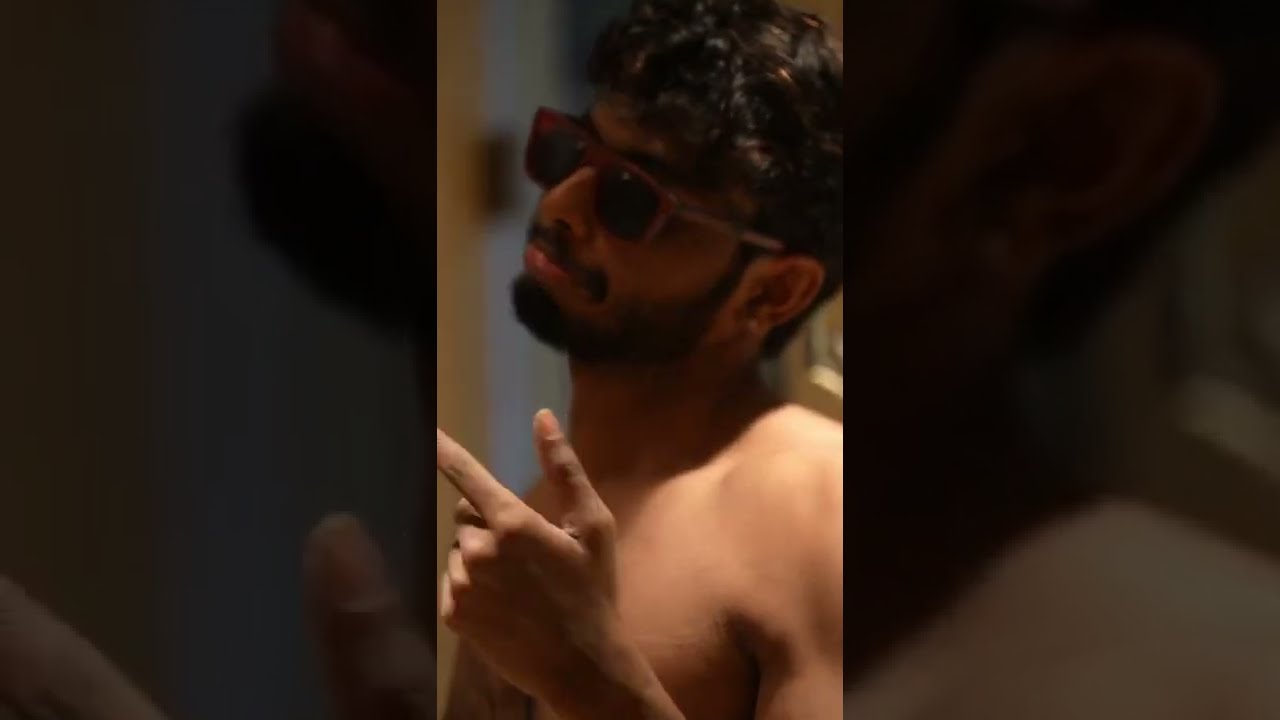The photograph captures a young man of Indian descent, shirtless, sporting a full beard and mustache. His short, wavy black hair is styled back and sits above his ears. He is wearing tan sunglasses with dark lenses and is positioned slightly turned to the left. The image is framed from his chest upwards, and he is holding his left hand up to his chest level, pointing his finger with his thumb slightly extended, reminiscent of a pistol gesture. He appears to be indoors, possibly near a window, as suggested by the light differences and the slightly blurry beige and white-toned background. Behind him, there is a hint of an open doorway contributing more light and the partial presence of a frame behind his left shoulder. The periphery of the image is tinted darker, giving a smoky effect and emphasizing the central part of the photo.